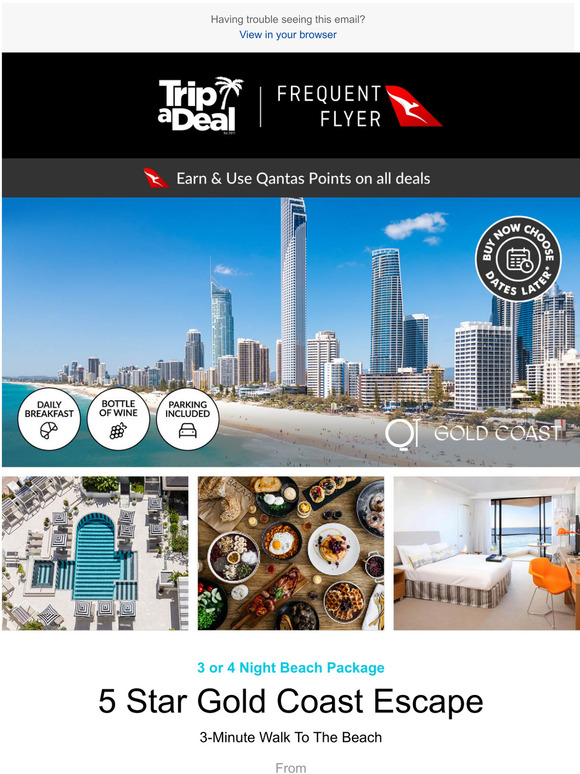The flyer prominently features the title "Trip A Deal" with the subtitle "Frequent Flyer." Beneath, it reads: "Earn and use Qantas Points on all deals." The main image showcases a stunning city skyline juxtaposed against water, with modern skyscrapers, a vibrant blue sky, and thin white clouds. Below this central image are three smaller pictures. The first shows a sleek, modern pool lined with numerous deck chairs. The second is a top-down shot of a table laden with a variety of breakfast foods, including finely plated eggs, an egg in a bowl, cut bread on a board, and waffles. The final image features a luxurious hotel room with a pristine white bed, a chair, and a window offering a view of the water. The flyer highlights a special offer: "4-night beach package at the 5-star Golden Coast."